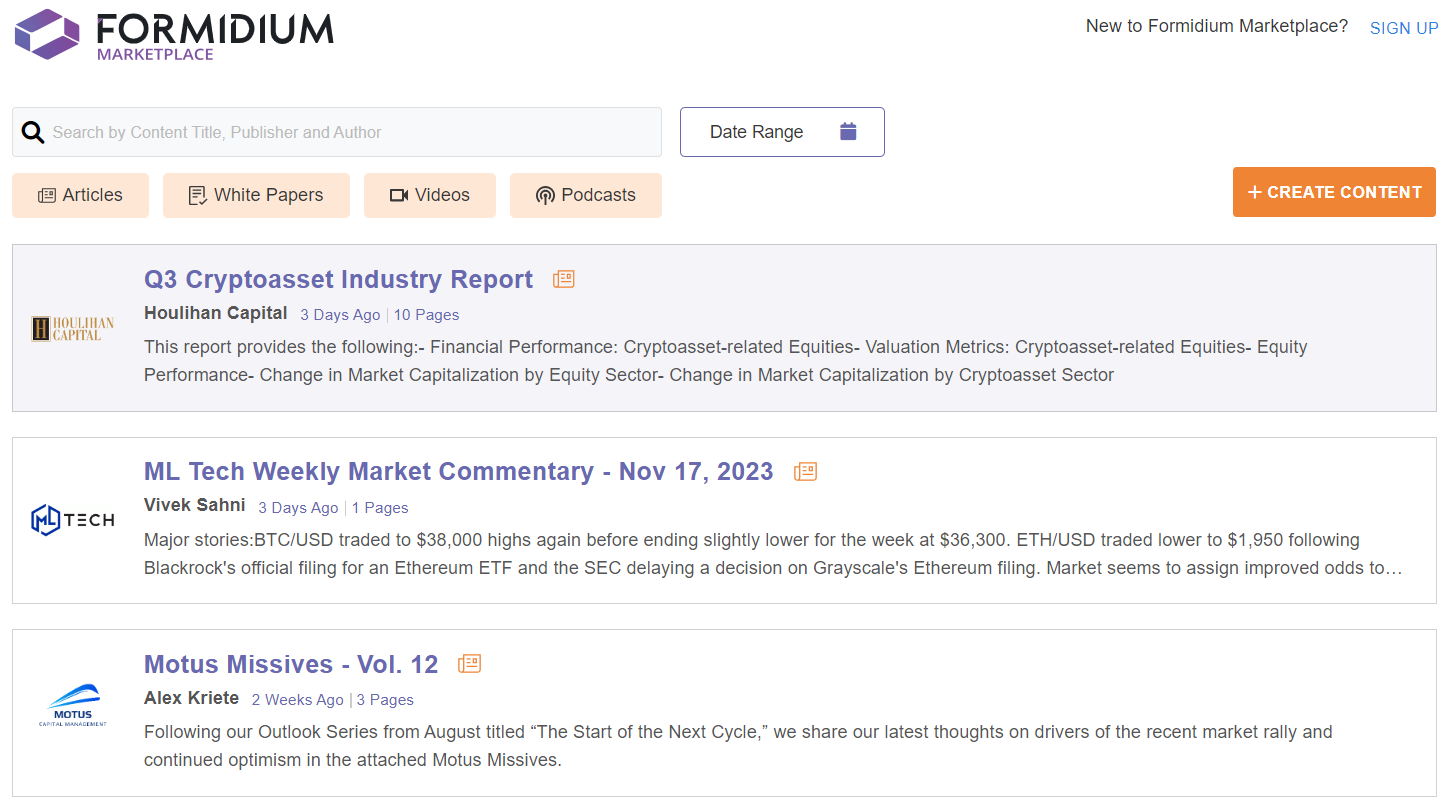Screenshot from the Formidium Marketplace interface:

The top section showcases the Formidium Marketplace header, where "Formidium" is displayed in black and "Marketplace" in purple, accompanied by a distinctive logo— a white diamond surrounded by four borders.

To the right of this header, a blue "Sign-Up" button is prominently featured beneath the text "New to Formidium Marketplace?"

Below the header, a search bar is present with placeholder text, "Search by content title, publisher, and author," available for filtering by date range and content type (articles, white papers, videos, and podcasts). An adjacent orange button allows users to "Create Content."

The main section lists three reports:

1. **Q3 Crypto Asset Industry Report** 
   - Published by: Houlihan Capital
   - Date: Three days ago
   - Length: 10 pages
   - Logo: Houlihan Capital logo
   - Additional details provided.

2. **ML Tech Weekly Market Commentary, November 17, 2023**
   - Author: Vivek Saini
   - Date: Three days ago
   - Length: 1 page
   - Logo: ML Tech logo
   - Additional details provided.

3. **Moto’s Missives, Volume 12**
   - Author: Alex Creti
   - Date: Two weeks ago
   - Length: 3 pages
   - Logo: Moto’s Missives logo
   - Additional details provided.